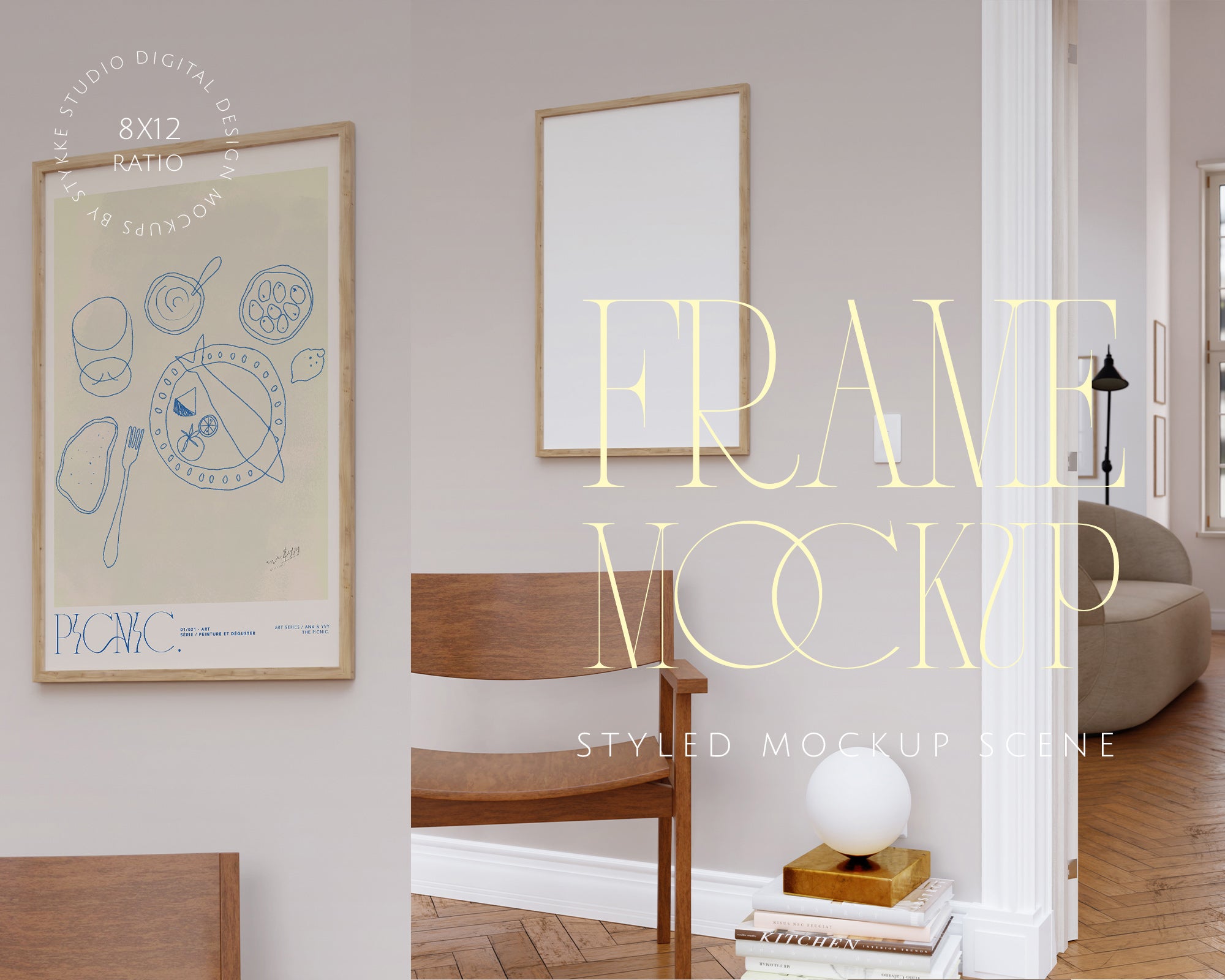This visually compelling design mock-up features a minimalist apartment interior with watermarked text that reads "frame mock-up, styled mock-up scene" and "studio digital design mock-ups by Stykke" set in a circular design with an 8 by 12 ratio indicated. The room’s herringbone wood floors complement its beige-gray walls and white trim, exuding a modern yet traditional vibe. In the foreground, a wooden chair is positioned next to a stack of books topped with an orb encased in a brassy base. On the wall above the chair, an empty wooden frame awaits personalization. Beyond this frame, a split-screen design reveals a portion of another frame containing minimalist line art depicting a picnic scene, including a plate with a fish, fruits, a fork, and a glass, illustrated in blue on a cream background. Through the doorway, more of the angled wooden flooring is visible, leading into another room furnished with a gray chair and a black floor lamp, further accentuating the apartment's chic simplicity. Empty wooden photo frames adorn the walls, maintaining the consistent minimalist aesthetic.